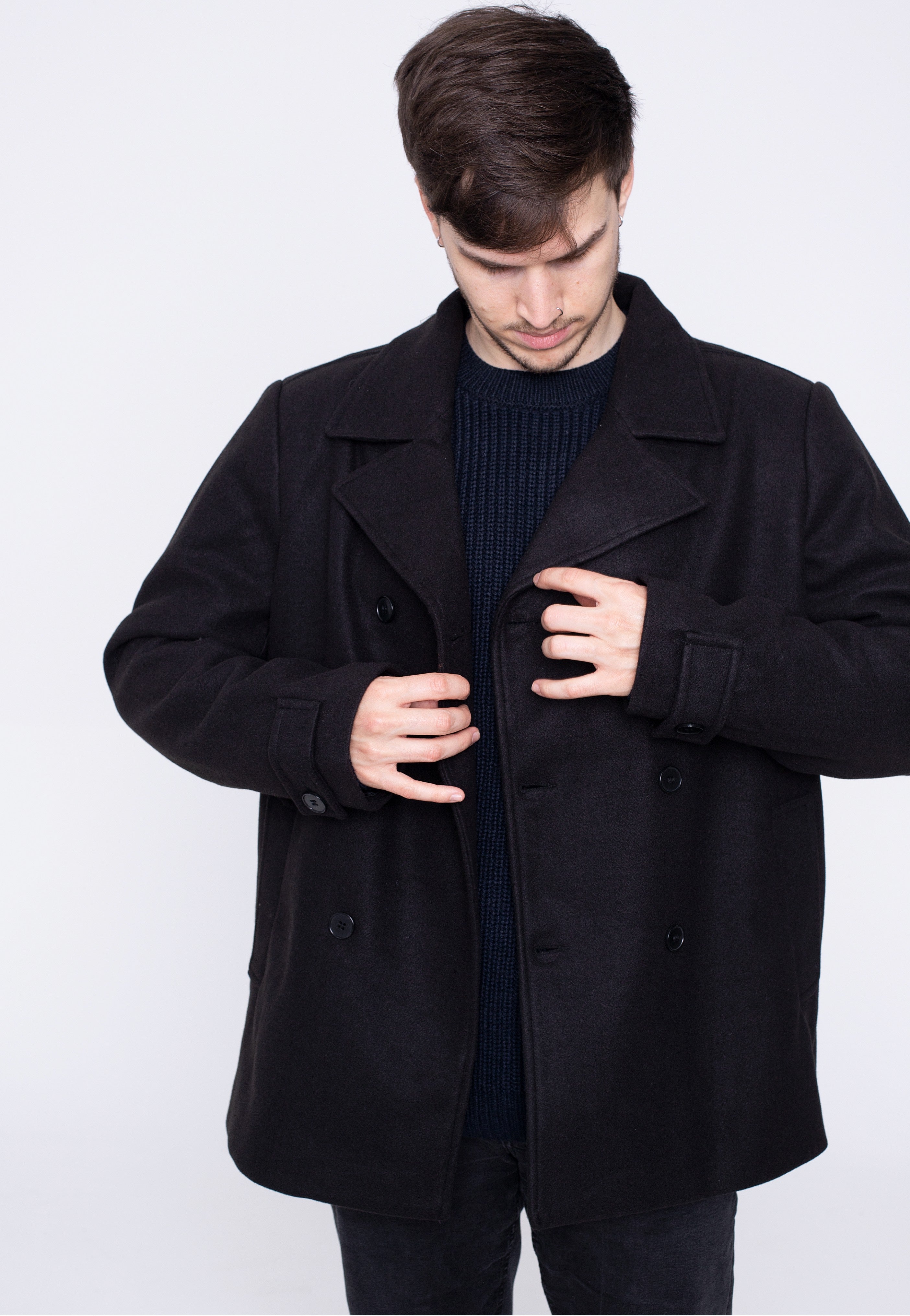A young Caucasian man in his 20s or 30s stands against a light gray or white backdrop. He has short dark brown hair parted to the side, dark eyebrows, and some facial hair including a mustache and goatee. He is dressed in a navy cable knit sweater under a slightly oversized, double-breasted black wool jacket with large lapels. The jacket features buttons on the front and straps on the cuffs. He appears to be adjusting or buttoning the jacket, looking down intently at his hands as they grasp the lapels. The man's outfit is completed with dark jeans. The overall demeanor suggests he is focused on his task, with the coat's longer sleeves creating a somewhat oversized appearance.